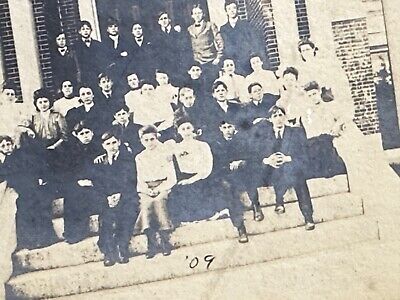This very old, black and white photograph appears to be from 1909, as indicated by the handwritten notation "’09" at the bottom. The image, which has a faded quality, features a group of approximately 20 to 30 teenagers, likely middle school to high school age, posing on the steps of a brick building, possibly a school or library. The group is arranged in four rows—boys standing in the back rows, and both boys and girls sitting on the staircase steps. The students are dressed in vintage early 1900s attire, with the males in suit jackets and ties, and the females in dresses. The photograph is marked by its serious tone, as none of the individuals are smiling, all gazing directly at the camera. The staircase they are sitting on leads up to a door that is obscured by the assembled group.